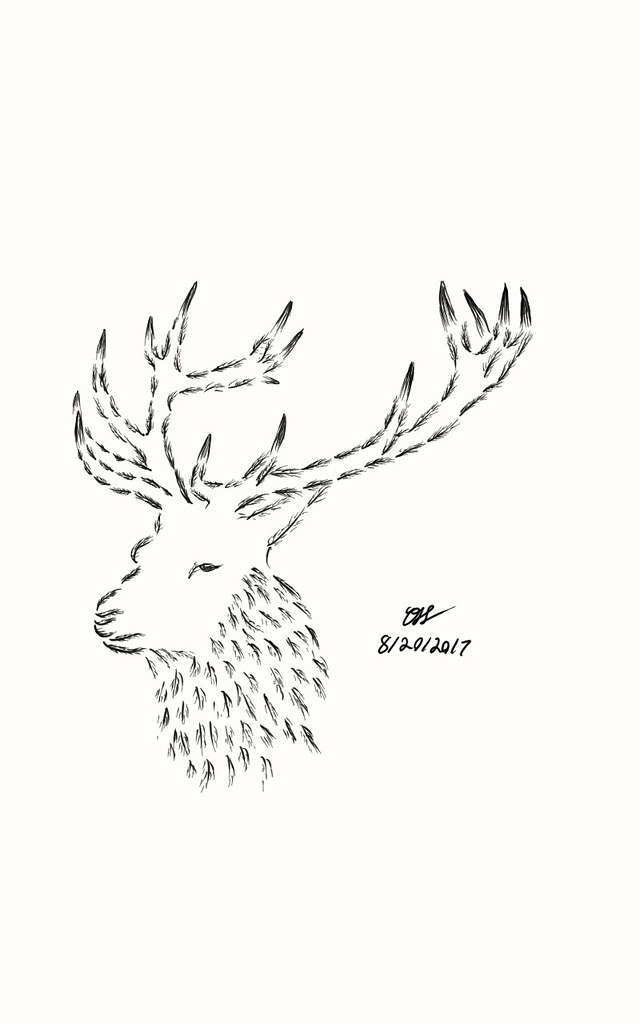This is a detailed pencil sketch of a deer, meticulously drawn against a white background. The deer is illustrated with fine pencil marks, giving it a textured and lifelike appearance. Its prominent antlers are adorned with subtle fur-like details, adding a touch of realism. The deer is depicted from an angled side view, showcasing its left eye, which appears gently closed. The artist has carefully rendered the neck with a series of lines that replicate the natural flow of the deer's hair. This thoughtful detail extends down its neck, enhancing the overall lifelike quality of the drawing. The artwork is signed in the bottom portion of the white background, with the date "8-20-2017" alongside the artist's initials. The deer's head is the focal point, crowned by notably large antlers that draw immediate attention.